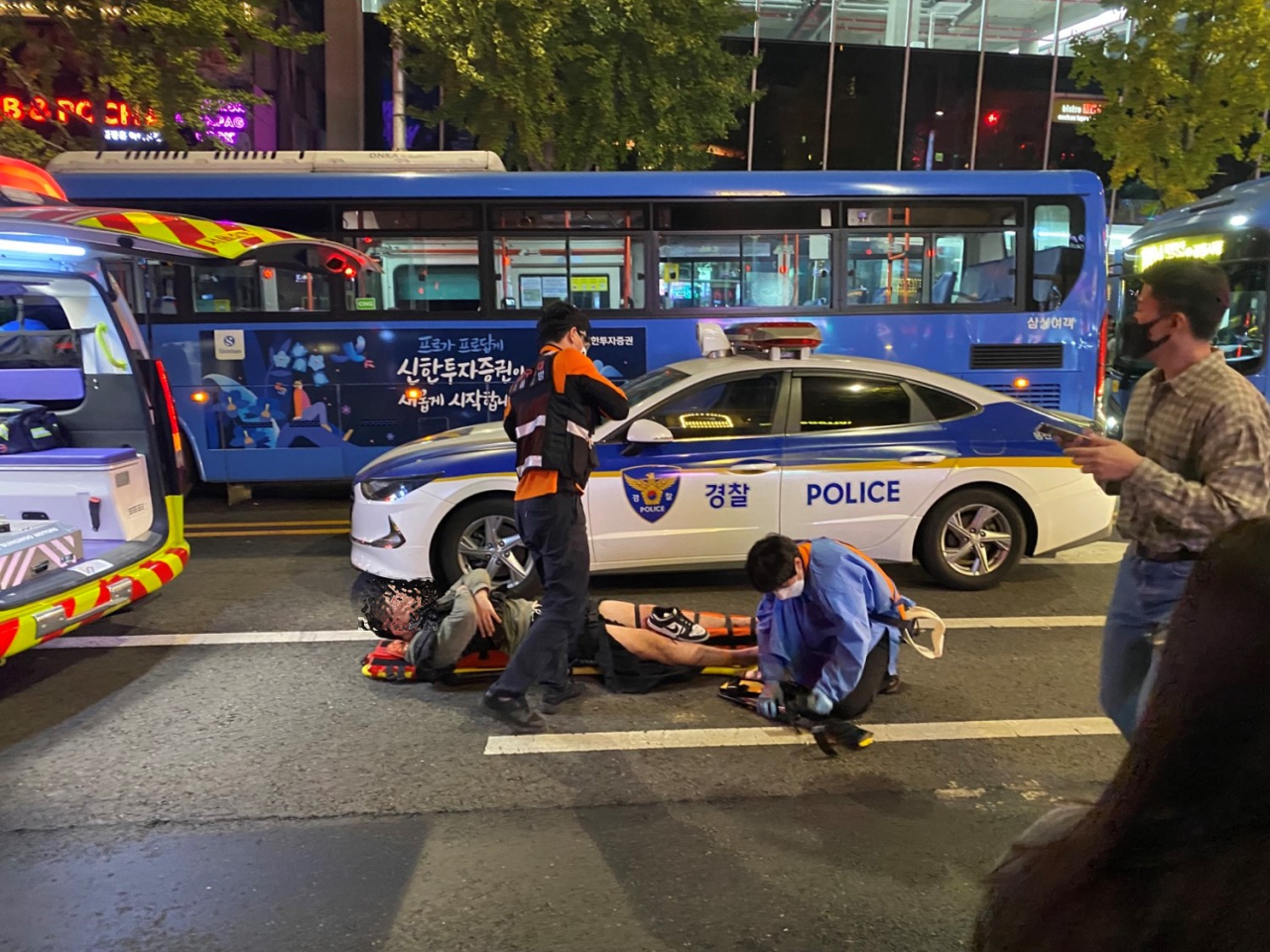This photo captures a dramatic scene on a bustling city street where emergency responders are attending to a man who has seemingly been involved in an accident. At the forefront, a man lies on a stretcher with his arms folded and a stabilizer affixed to his left leg. His athletic shoe rests between his legs, possibly removed to allow medical treatment. Two paramedics are diligently working: one, dressed in a black and orange emergency jacket, stands while overseeing the situation, and the other, wearing a blue sweatshirt and blue gloves, kneels and manages medical equipment. Both are masked, emphasizing the ongoing safety protocols.

To the left, the open back of an ambulance with its interior seats visible hints at the urgency of the situation. A white police car with red and yellow trim and an emblem featuring an eagle on a badge is stationed behind the stretcher, displaying both English and oriental characters on the driver's side door. Its red lights flash, underscoring the severity of the moment. Further back, a blue city bus marked with oriental writing stands still, perhaps halted by the ongoing emergency, its absence of passengers notable.

A bystander in jeans and a brown-striped shirt, masked and engrossed in his phone, walks past the scene to the right, casting a glance at the unfolding drama. The overall scene conveys a snapshot of a city's emergency response, complete with the vivid details of uniforms, vehicles, and the calm amidst a tense and urgent situation.